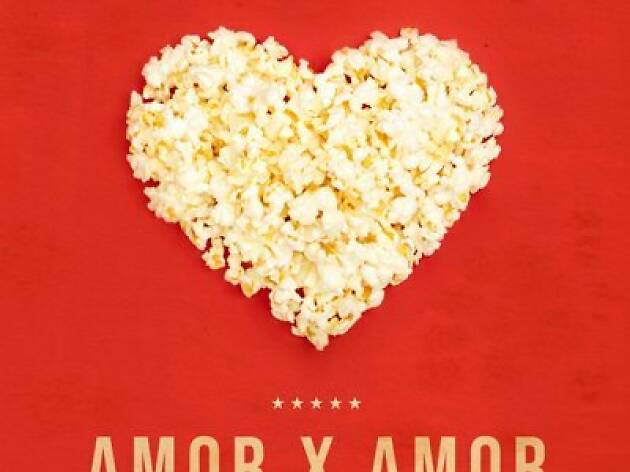The image features a vivid red background that dominates the scene. At the center, stretching from the top to slightly below the midpoint, is a heart shape constructed from fully popped popcorn kernels in shades of yellow and white. Directly below the heart, in the middle of the image, are five small stars that share a similar tan color to the popcorn. Further down, at the very bottom of the image, there is text displayed in a large, capitalized font. The text appears to read "A-M-O-R," followed by a space, an ambiguous letter that looks like an 'X,' and again "A-M-O-R," although it's partially cut off and not entirely clear.